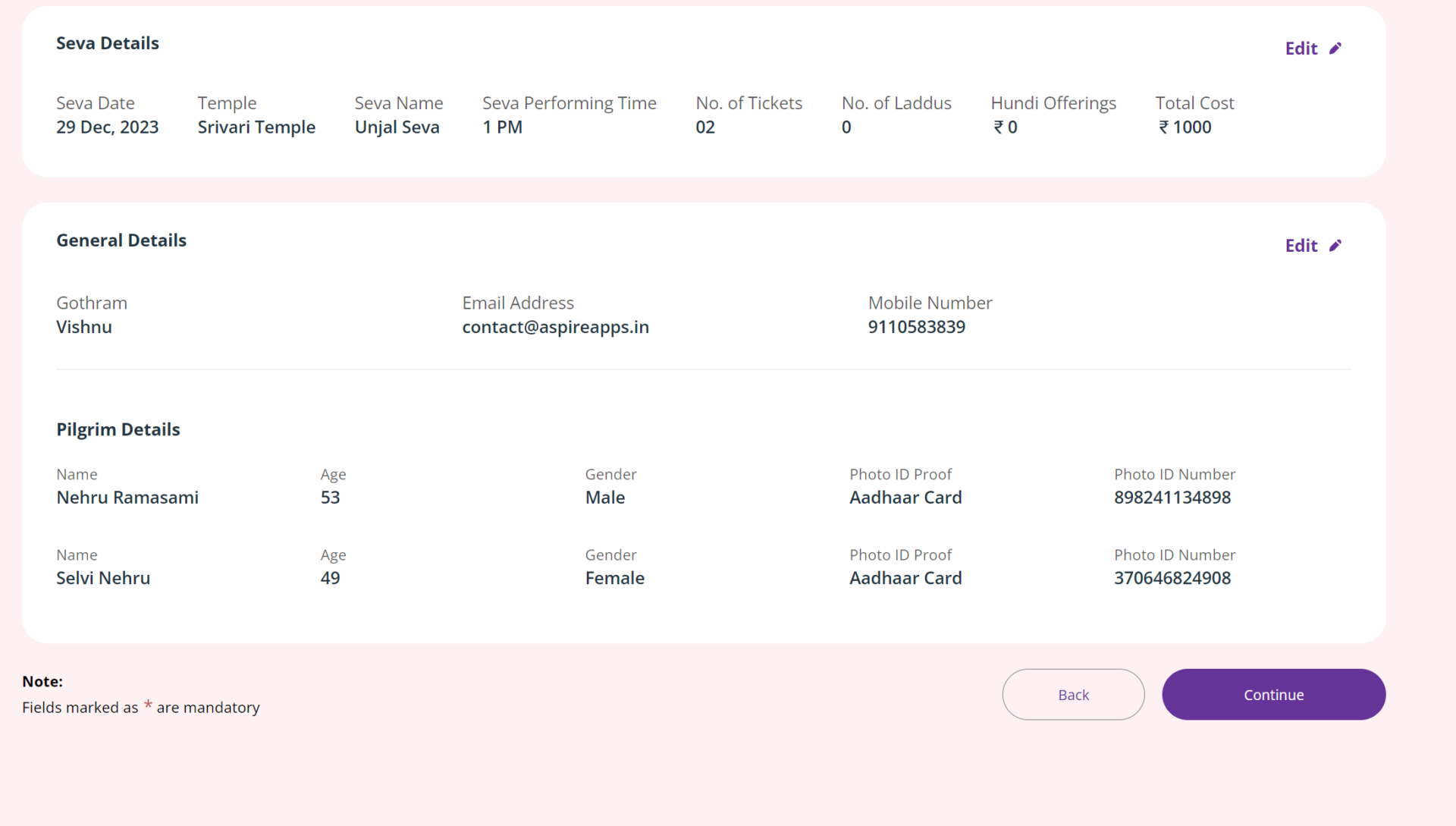Screenshot of Save Seva Details:

The screenshot features a user interface with a light pink square background. Two overlaying boxes organize the details. The first, smaller box is white and includes several fields: 

- **Seva Date**
- **Temple**, specifically “Serebii Temple”
- **Seva Name**
- **Seva Performing Time**
- **Number of Tickets**
- **Number of Lattice**
- **Hyundai Offerings**

Following these fields is the total cost displayed as "$1,000 in Hindu currency."

The larger box below is labeled "General Details" and includes:

- **Name**
- **Email Address**
- **Phone Number**

It is followed by "Pilgrim Details" which captures:

- **Name**
- **Age**
- **Gender**
- **Photo ID and Photo ID Number**

Details for a second guest include:

- **Age: 49**
- **Gender: Female**
- **Proof of ID and Photo ID Number**

Below these entries, a note indicates that some fields are mandatory. 

At the bottom of the interface are two buttons: a gray-outlined "Back" button and a solid purple "Continue" button in white text.